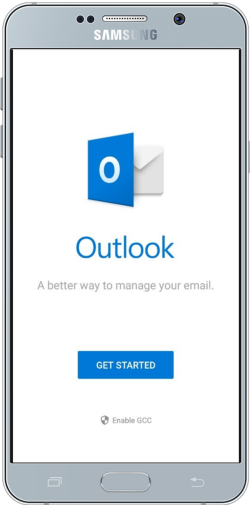The image showcases a gray Samsung cell phone with a focus on its sleek design and the display screen featuring the Outlook application. The phone is centrally positioned in the frame, highlighting its minimalist aesthetic. The Samsung logo, which is rendered in a light, mirror-like font, is placed just below a thin speaker grille at the top of the device. To the left of the speaker are two small sensor holes, while on the right side, a larger hole is visible, likely housing the front-facing camera.

Along the left edge of the phone, the volume up and down buttons are subtly visible, adding to the functional elements of the device. The display screen is currently showing the Outlook app, which is predominantly white and presents the Outlook logo prominently in the center. The logo consists of a stylized "O" block facing left, partially overlaying an envelope icon, symbolizing email. Below the logo, the word "Outlook" is displayed in a thin, blue font with a capital "O," maintaining the app's clean and professional appearance.